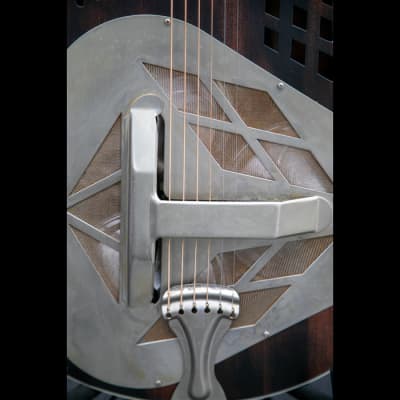This is a detailed close-up photograph of the inside of a guitar-like musical instrument, revealed with its face cover removed. The instrument features six strings, each anchored in designated holes visible in the image. The strings vary from thin on the right side to thicker gauge on the left, suggesting it might be an electric guitar. The body of the instrument appears silverish-gray in color, with a brown wooden base noted between what would be the air holes. The photograph highlights a metal structure within the instrument, resembling a capital T turned on its side, and attached to a triangular piece of metal. Some of the screws and face plating are missing, providing a unique view of the internal mechanics, including a bridge and possible cut polygonal and triangular patterns on the left side. The overall impression is of a deconstructed guitar, intricately detailed in its exposed form.